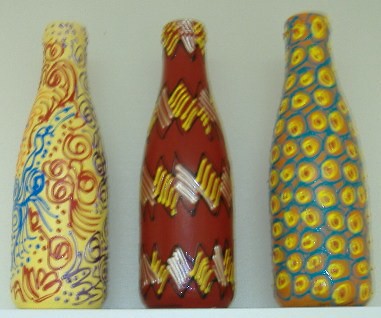This photograph captures three distinctively painted bottles, lined up side by side against a light gray backdrop. They are all the same size and shape, cylindrical and narrowing towards the top, with each one adorned in unique, vibrant patterns. 

The bottle on the left features a light yellow background, adorned with an energetic array of swirls, dots, and scribbles in shades of red, purple, and blue. The central bottle, set against a maroon or orangey-brown backdrop, boasts four horizontal bands of alternating yellow and white zigzags. These zigzag patterns create a dynamic visual effect as they run down the length of the bottle. The bottle on the right presents a primarily blue background, overlaid with a series of yellow circles, each having a darker center encircled by a blue ring. These circles repeat across the bottle, almost touching edge to edge, with the orange base color subtly showing through where the blue rings meet. All three bottles are oriented vertically and are set in a row, showcasing their bright, eclectic designs.